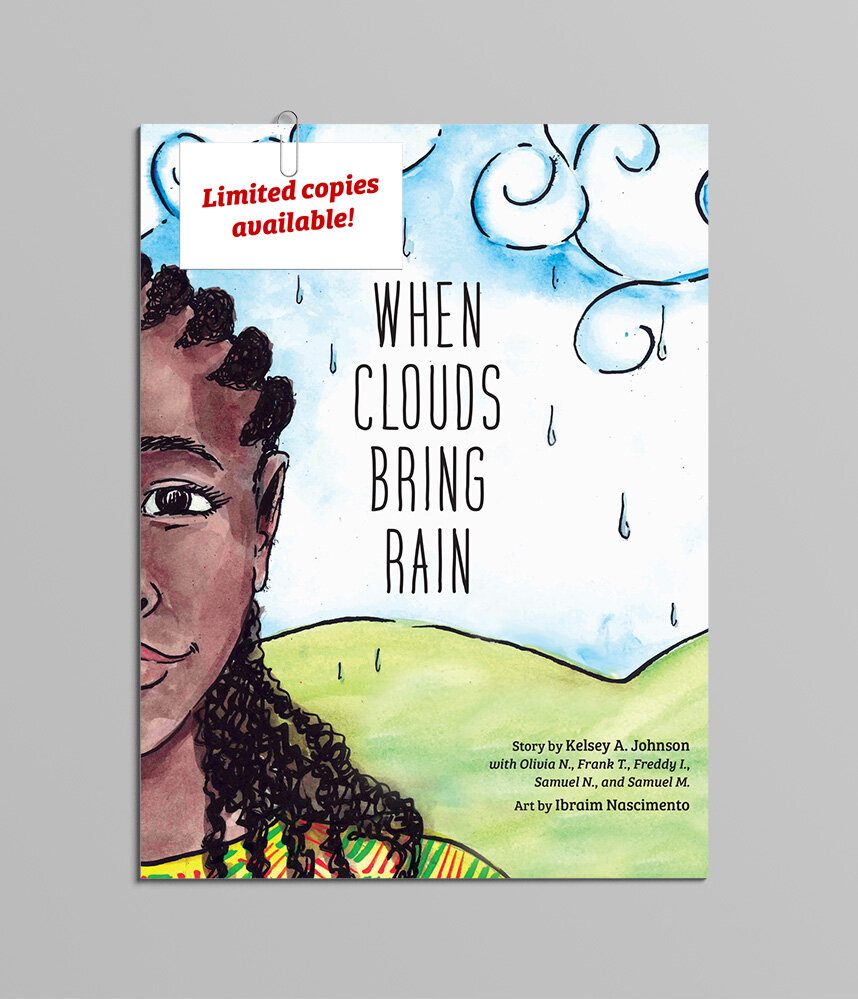The image depicts the cover of a book titled "Wind Clouds Bring Rain." Dominating the left side of the cover is a striking illustration of an African American woman with cornrows, though only the left half of her face is visible. She wears a shirt or jacket featuring a combination of green, yellow, and red colors. At the top left corner, a small card is paper-clipped, proclaiming in red text that there are "limited copies available." The background of the cover transitions from a blue sky filled with raining clouds to a scenic view of green rolling hills in the bottom third. Additional text on the cover indicates that the story is by Kelsey Ann Johnson, with contributions from Olivia R., Frank T., Freddie I., Samuel N., and Samuel M., and the art is credited to Abram Nacimenta. The composition expertly balances the portrait of the woman with the serene, evocative landscape.